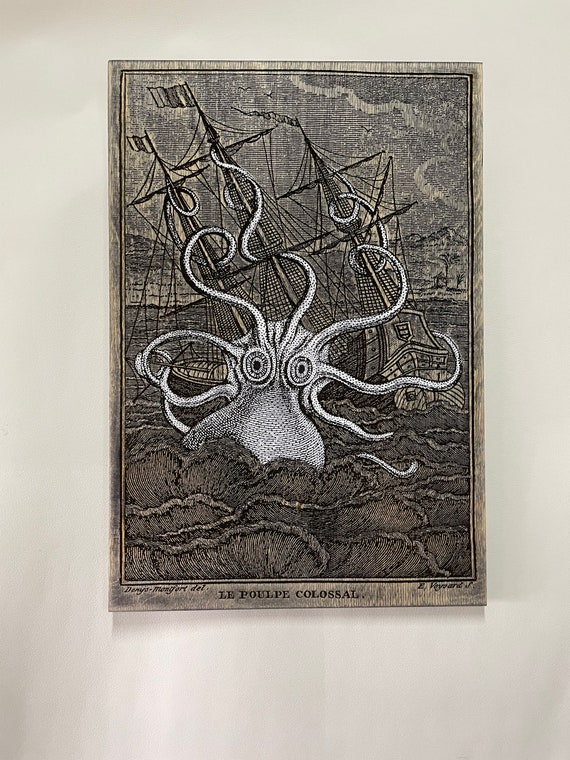This image depicts an intricate black and white artwork mounted on a gray-shaded wall, suggesting it is an older piece. The primary focus of the drawing is a colossal white octopus, with its massive tentacles intertwined around a large sailing vessel, almost overshadowing the ship. While part of the octopus's head remains submerged underwater, its topmost tentacle nearly reaches one of the masts, highlighting its immense size. The sea around the ship appears choppy, adding to the dramatic effect of the scene. The sky in the background looks stormy, enhancing the ominous atmosphere. Inscribed at the bottom of the drawing are the words "Le Poulpe Colossal," translating to "The Colossal Octopus." Additional script flanks the title, although it's too small to discern. A signature, presumably the artist's, is etched at the bottom, solidifying its authenticity.